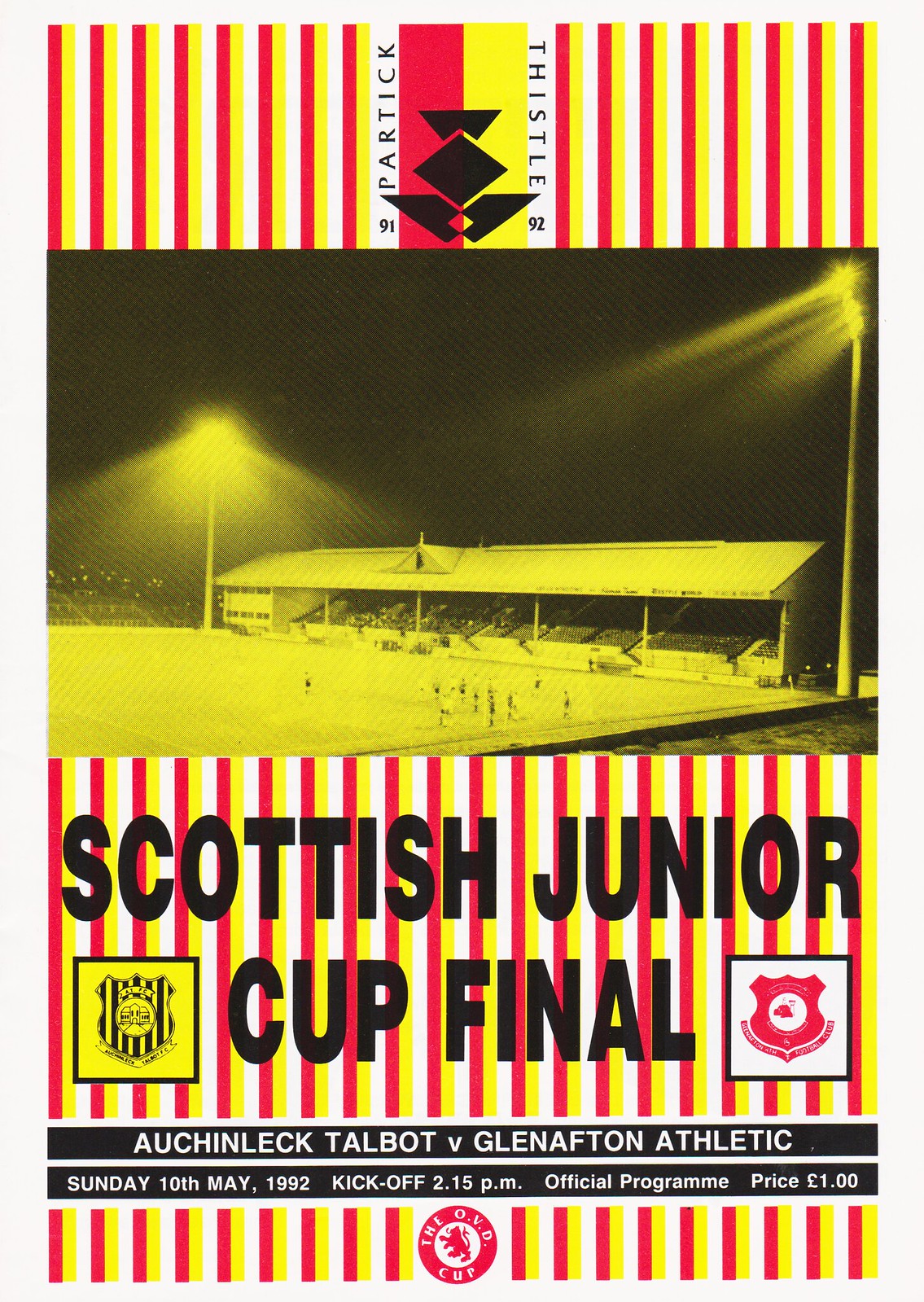The image portrays an advertisement for the Scottish Junior Cup Final, prominently featuring red, yellow, and white vertical stripes as its background. At the top center, there’s a logo displaying the numbers "91" and "92" with the words "Patrick Thistle" split on either side. Below this, a black-and-white, dusk-time photograph of a stadium reveals blurry figures on the field, illuminated by large floodlights with visible stands. The central text reads "Scottish Junior Cup Final," flanked by team crests: a yellow-and-black emblem on the left and a red-and-white emblem on the right. Below this, a black bar contains white text stating, "Auchinleck Talbot v Glen Afton Athletic." Another black bar beneath it announces, "Sunday, 10th May 1992, kickoff 2:15 PM, official program price £1." At the very bottom, a red and white logo for the "OVD Cup," featuring a lion or bull, completes the design.